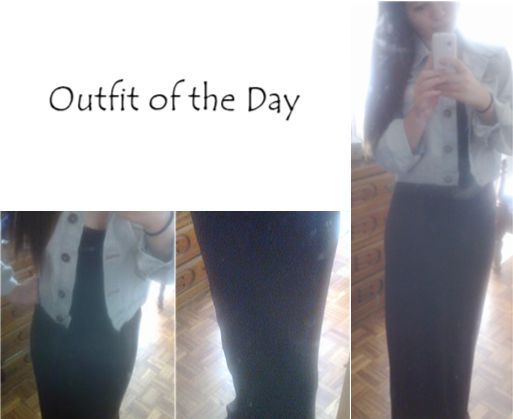This is a collage of three images featuring a young Caucasian woman capturing her outfit of the day. The central image on the right showcases her full body, where she wears a long black dress paired with a light denim jacket cuffed at the elbows and left unbuttoned. Her dark hair cascades over her shoulder as she holds a white phone in front of her, taking a mirror selfie. A bracelet is visible on her right arm. The floor beneath her is a brown parquet, and a brown dresser stands behind her, contributing to a candid atmosphere with imperfect lighting and noticeable glare.

To the left of this full-body photo, the phrase "outfit of the day" is printed in black text on a white background. Below this text, the collage features two additional images: one depicts her midsection, highlighting the denim jacket over the dress, and the other shows the hem of the dress touching the wooden floor. Despite the overall blurriness and glare affecting the photo quality, the collage effectively details her attire.